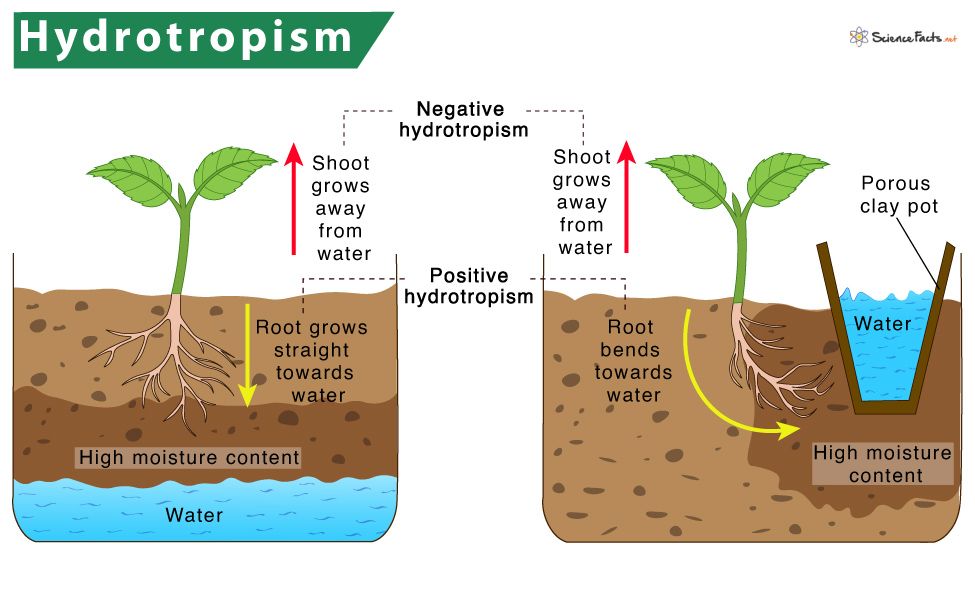This is a scientific cartoon diagram titled "Hydrotropism," displayed in white text on a green banner at the top right. The diagram, sourced from an educational website (sciencefacts.net), illustrates the concept of hydrotropism through two side-by-side cross-sectional images of soil and plant growth. 

In the left image, we see a land cutout resembling a beaker containing a small sprout. The roots grow straight down towards the high moisture content area labeled as "water" at the base. An accompanying arrow and text state, “root grows straight towards water below,” emphasizing positive hydrotropism. The plant shoot grows away from the water, indicated by an upward arrow.

In the right image, another small plant is shown with roots that bend towards a nearby water source contained in a porous clay pot buried in the soil. The arrow next to the roots is labeled "root bends towards water," also denoting positive hydrotropism. Above the pot, a black font states "water," with darker soil around the roots marked as "high moisture content." Again, an arrow indicates that the plant shoot grows away from the water.

This detailed diagram visually differentiates between positive and negative aspects of hydrotropism, focusing on the roots' behavior in seeking water while the shoots grow away from it.